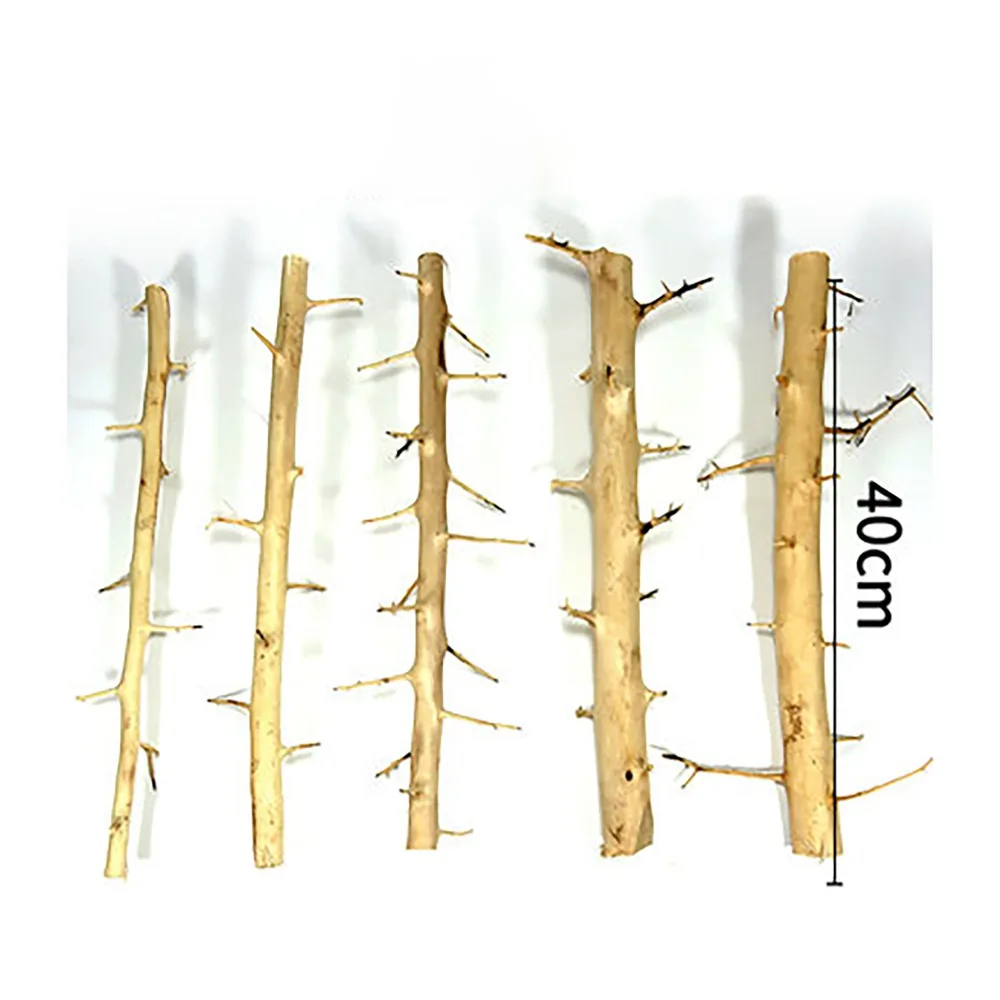In this image, we see five thin, bare segments of potentially a rosebush laid out on a white or off-white background. Each branch is light brown, with some getting darker toward the top, and they have smaller, twig-like branches protruding from the main stalk. The branches appear progressively thicker from left to right. The first branch has around six to seven smaller branches, the second about eight, with the central branch having a few more and slightly thicker ones. The two on the right are noticeably thicker in diameter and also feature smaller branches. All five segments cast visible shadows, which become more pronounced with the thicker branches. A black measurement scale on the right-hand side marks the length of these segments at 40 centimeters, providing a sense of their size. The appearance of the branches suggests they have been bleached, either by sunlight or chemically, giving them a pale, blonde hue.